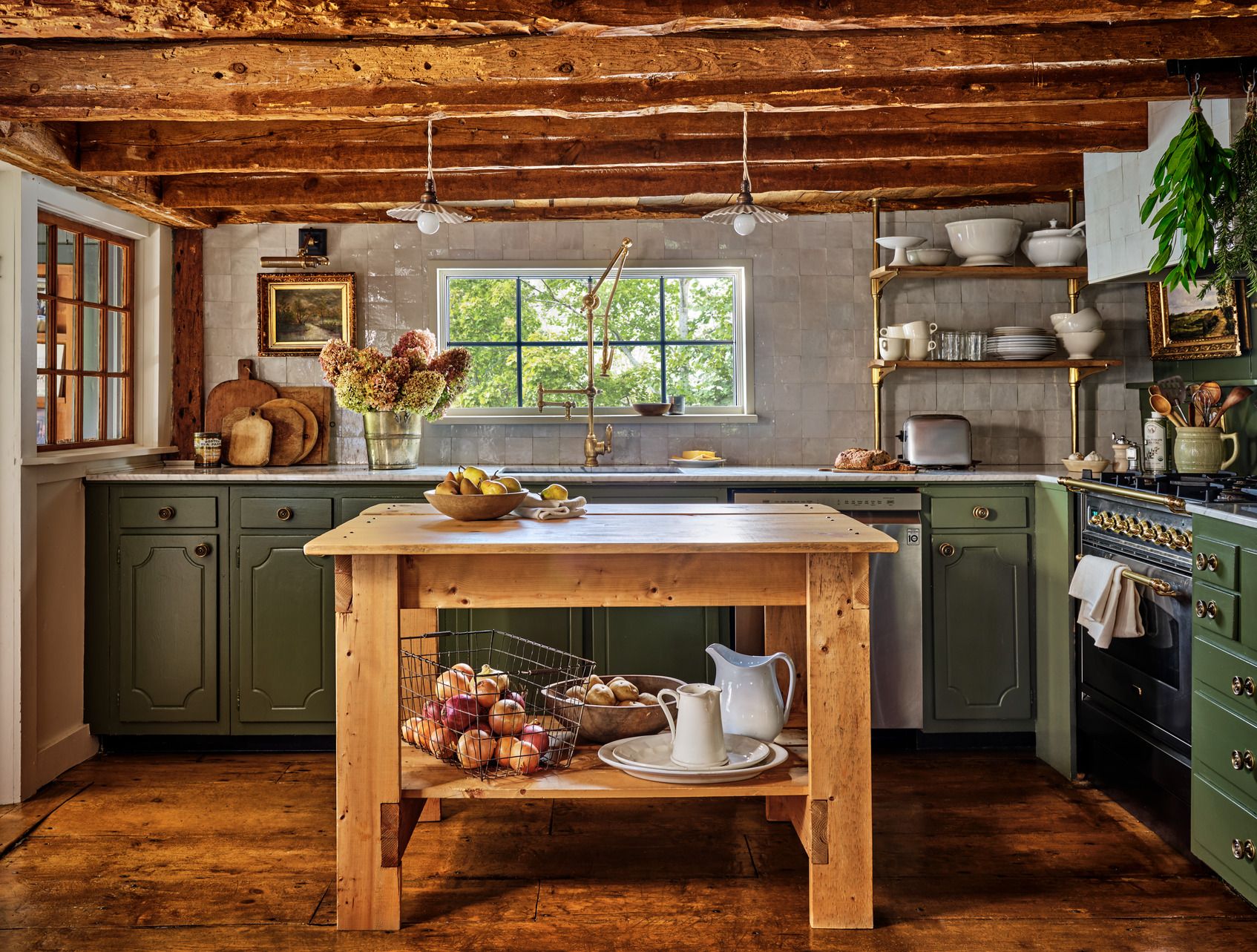The image depicts a rustic country kitchen enveloped in an old-world charm. The ceiling features aged, rough-hewn wooden beams in hues of brown and yellow. Suspended from these beams by two strings is a light bulb fixture. The back wall, built of slender gray bricks, hosts an eight-pane window revealing the greenery outside, allowing natural light to stream in. To the left of the window, a painting hangs above a vase adorned with flowers and wooden cutting boards. To the right, open shelves made of metal rods and wood slats house white pots and a metal toaster beneath, while a black stove with golden handles stands nearby. Green-painted cabinetry with metal handles lines the walls, topped with white countertops. In the center of the kitchen, a sturdy wooden island stands tall, matching the countertop height. The island's top holds a bowl of pears, while its lower shelf contains baskets with apples and possibly potatoes, along with white ceramic pitchers for liquids. The floor is a worn but smooth wood, enhancing the room's rustic feel. To the left, a doorway begins, flanked by another window. Decor elements like greenery hanging from the ceiling and a ceramic crock filled with wooden spoons on the stove contribute to the kitchen’s vintage allure.